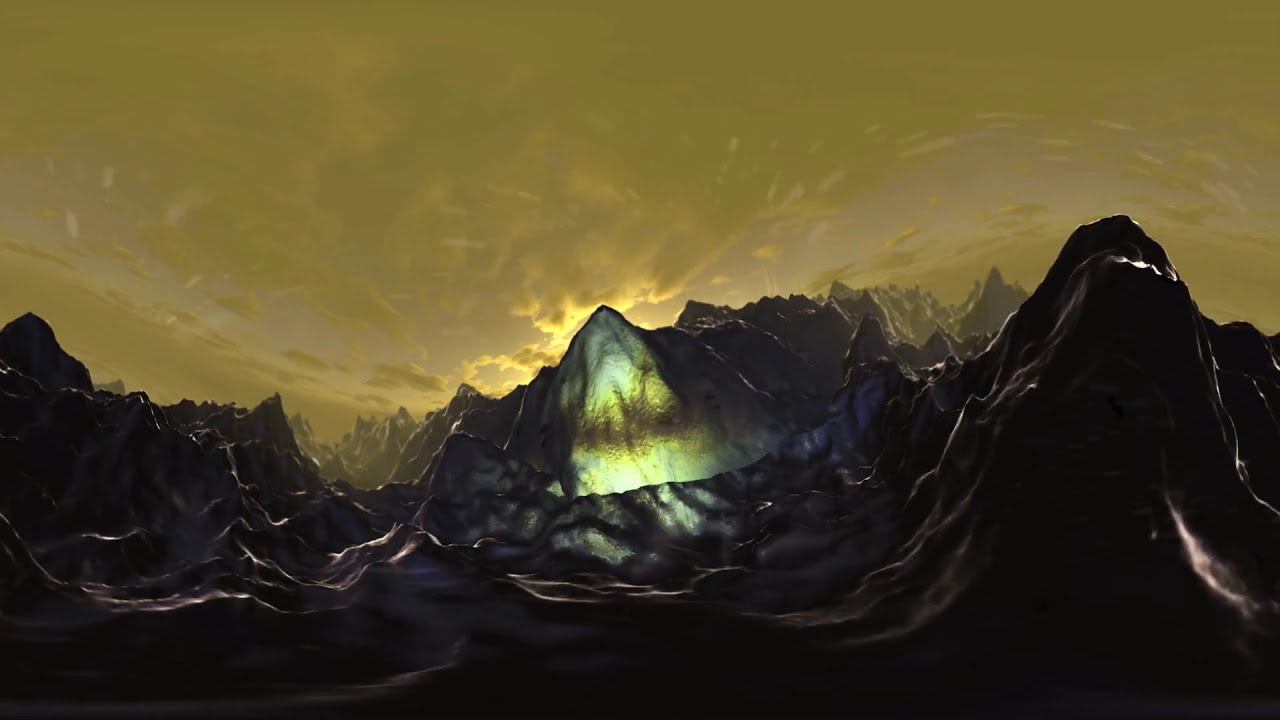The image depicts a surreal, almost otherworldly landscape that appears computer-generated. It features craggy, barren mountains dominating the bottom half, with dark tones of black, grey, and hints of purply-blue. The mountain range is characterized by sharp, jagged peaks, some resembling a set of sharp teeth, and a larger, more rounded peak on the right. In the middle of the image, another mountain range rises, with a glowing center in shades of light green, yellow, and brown, as if illuminated from within. Above, the sky is a swirling mix of golden yellow, with streaky clouds accumulating, some in grayish-green hues, creating a dramatic, desolate atmosphere. The overall effect is a stark, textured, and vividly colored landscape that seems alien and otherworldly.